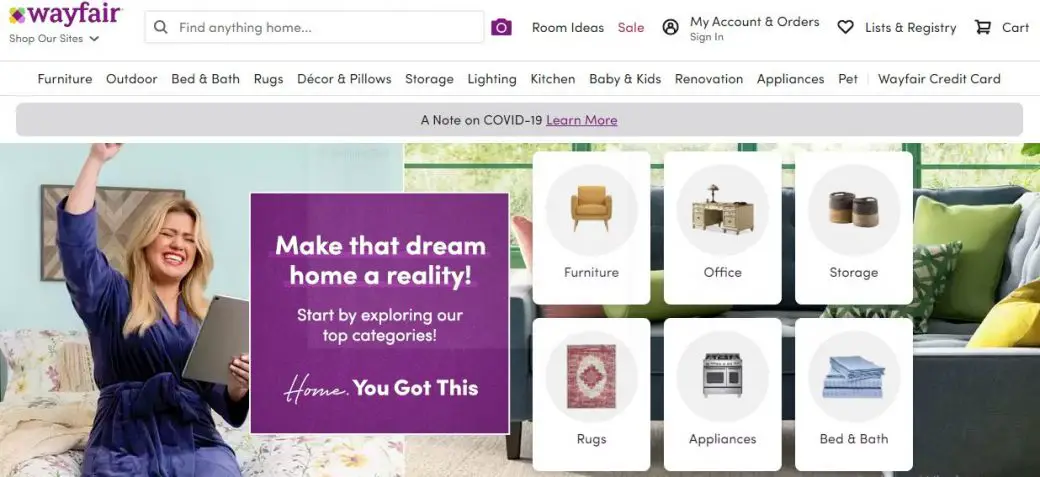This is a detailed screenshot of the Wayfair website, prominently displaying its user interface elements and layout. At the top left corner, the website's name, "Wayfair," is featured in a distinct purple font alongside its recognizable logo. Directly below, there’s an option labeled "Shop Our Sites" with a dropdown arrow, facilitating easy navigation to different areas of the site. 

To the right of this, there is a search box with the placeholder text "Find anything home," allowing users to input search queries. Adjacent to the search box, there’s a purple camera button for search by image functionality. Continuing to the right, several navigation links are present: "Room Ideas," "Sale" (highlighted in light purple), "My Account," "Orders," and "Sign In." Further right, links for "Lists and Registries" and the "Cart" icon finish off the top navigation bar.

In a secondary navigation layer beneath, there are categorical links: "Furniture," "Outdoor," "Bed & Bath," "Rugs," "Decor & Pillows," "Storage," "Lighting," "Kitchen," "Baby & Kids," "Renovation," "Appliances," "Pet," and "Wayfair Credit Card." This categorical navigation ensures users can delve deeper into specific areas of interest.

A gray banner below these links contains a note on COVID-19 with a purple hyperlink that reads "Learn more," providing additional information about the company's handling of the pandemic.

The main visual content includes a left-aligned image of Kelly Clarkson, who is joyously pumping her right fist into the air, eyes closed and smiling, suggesting she has received a great deal. To the right of her image is a prominent purple box, outlined in white, with the motivational text "Make That Dream Home a Reality." Below this, in white font, the text reads, "Start by exploring our top categories. Home, you got this."

Adjacent to this text, three columns feature different categories with thumbnail images of representative items. The categories include "Furniture" (displaying an easy chair), "Office" (featuring a desk), "Storage" (showing various storage solutions), "Bed & Bath" (illustrating a sheet set), "Appliances" (depicting a stove), and "Rugs" (showing a rug), guiding users visually through different product offerings.